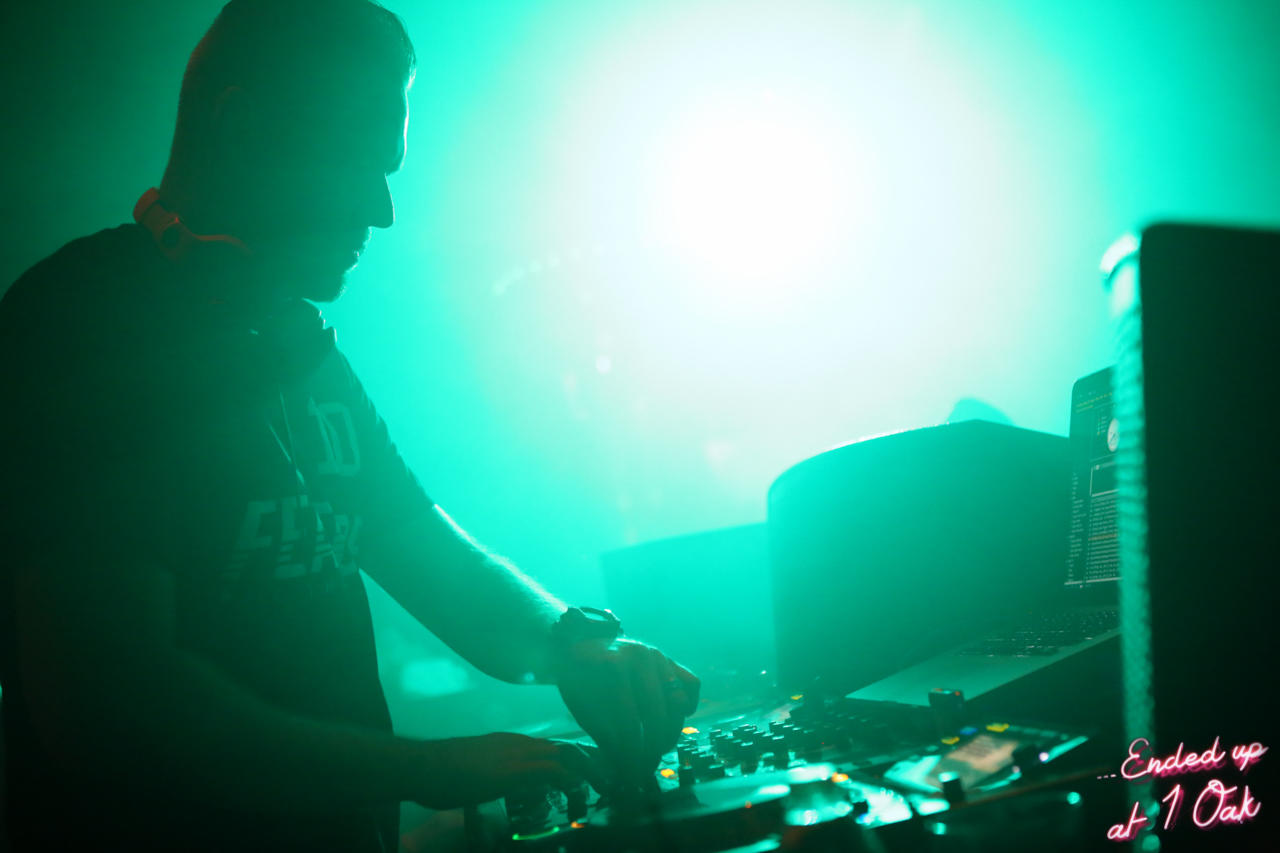This image captures the side profile of a man, likely a DJ, who is deeply engaged with his equipment, situated in a club environment. He's seen facing to the right, looking down at what appears to be a turntable, turning its knobs with precision. He wears a short sleeve t-shirt with text on it, a watch on his left hand, and has a pair of headphones resting around his neck.

The overall scene is suffused with a neon teal light, casting a unique green-blue hue across the image. The light source is situated towards the center-right, creating a significant glare that dominates the background and blends into a bright white core. This adds a dramatic, almost ethereal ambiance to the photo, emphasizing the silhouette of the DJ.

In addition to the turntable, various pieces of sound equipment, including a laptop with its screen on, speakers, and control dials, are visible around him, indicating a professionally set up DJ booth. Despite the darkness of the room, these details are illuminated by the ambient club lighting, contributing to the vibrant atmosphere.

In the bottom right corner of the image, the phrase "ended up at one oak" is written in red script, providing a narrative touch to the scene. The overall mood of the photo is energetic and dynamic, capturing a moment of musical engrossment and club culture.